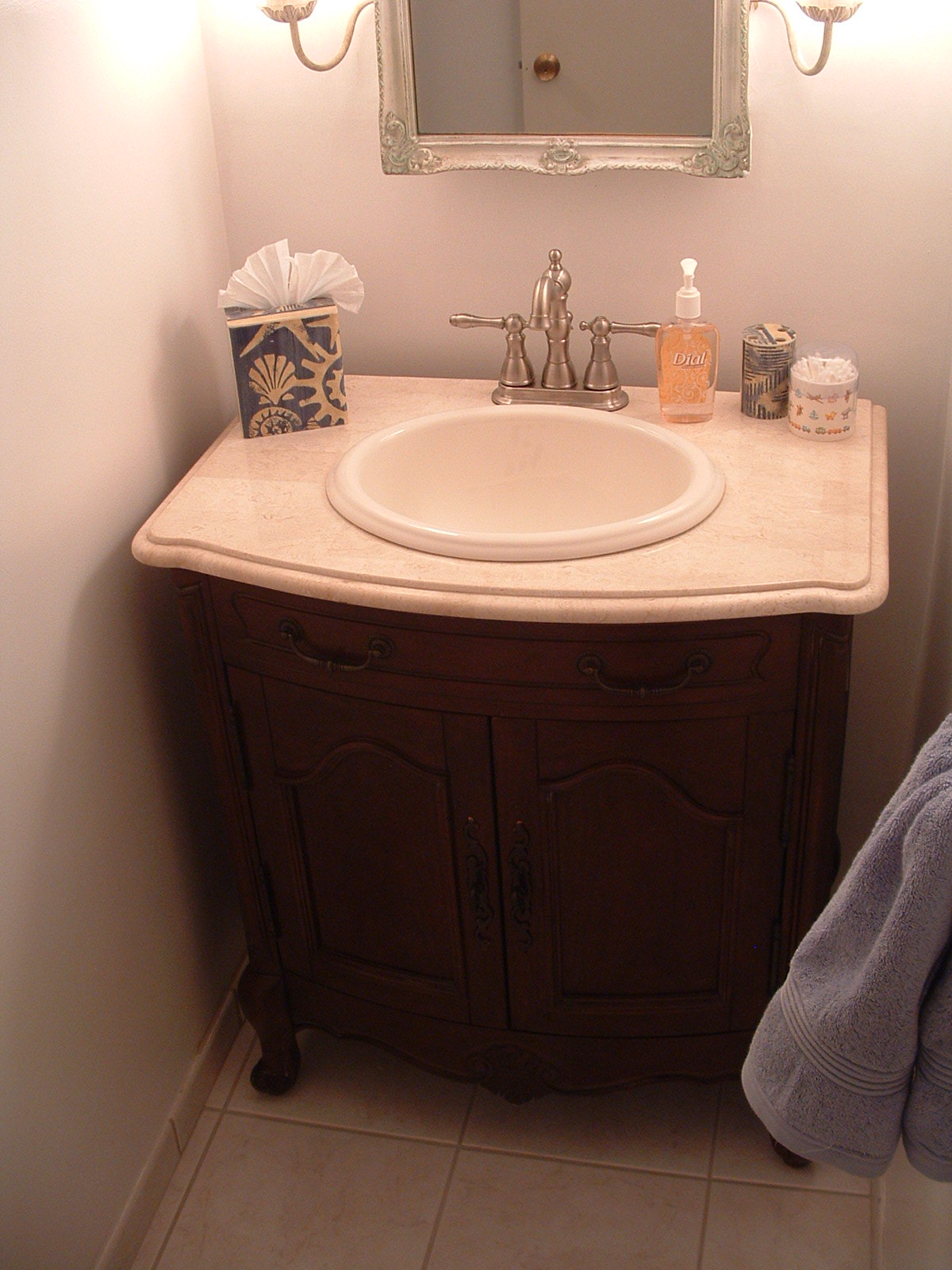This photograph showcases a neatly arranged bathroom corner featuring a stylish sink area. The bathroom floor is adorned with gray tiles that seamlessly blend with the pristine white walls. The sink, embedded in the corner where these two walls meet, sits elegantly atop a smooth, marble-esque countertop, characterized by its off-white to light tan hue. The centerpiece of this arrangement is a sleek, white oval sink accompanied by a silver water fixture that includes both a faucet and matching handles for precise control.

To the right of the sink, a bottle of Dial hand soap stands prominently, ensuring cleanliness at hand. Adjacent to it is a mysterious gray and yellow cylindrical container, the contents of which are not visible, adding an element of intrigue. A small cup filled with organized Q-tips completes the countertop accessories.

The base of the sink unit features two drawers and two cabinets constructed from very dark wood, creating a striking contrast against the lighter tones above. The cabinets' bent leg support elevates the entire unit, giving it a refined, classic appeal. In the foreground, a gray towel is neatly draped over a towel rack on the right-hand side, contributing to the overall sophisticated and well-maintained ambiance of the bathroom.